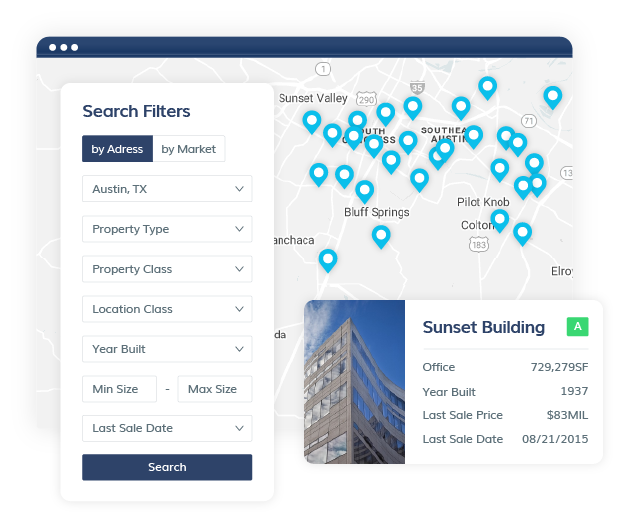The image is a screenshot of a location-based search interface. At the top of the screen, there is a dark blue banner with three white dots in the upper left corner. Below this banner, a light gray map with white roads is displayed, featuring several blue pins throughout key areas including Sunset Valley, Southeast Austin, Bluff Springs, and Pilot Knob. On the left side of the screen, a white sidebar contains search filters titled in bold black text with a highlighted blue accent. Within this sidebar, the options include two primary buttons: 'By Address,' which is currently highlighted, and 'By Market,' which remains unselected. Beneath these buttons are various filter options such as 'Austin, Texas,' 'Property Type' dropdown, 'Property Class' dropdown, 'Location Class' dropdown, 'Year Built' dropdown, 'Minimum Size' and 'Maximum Size' input boxes, and a 'Last Sold Date' dropdown. At the bottom of the filters, there is a prominent blue action button labeled 'Search.'